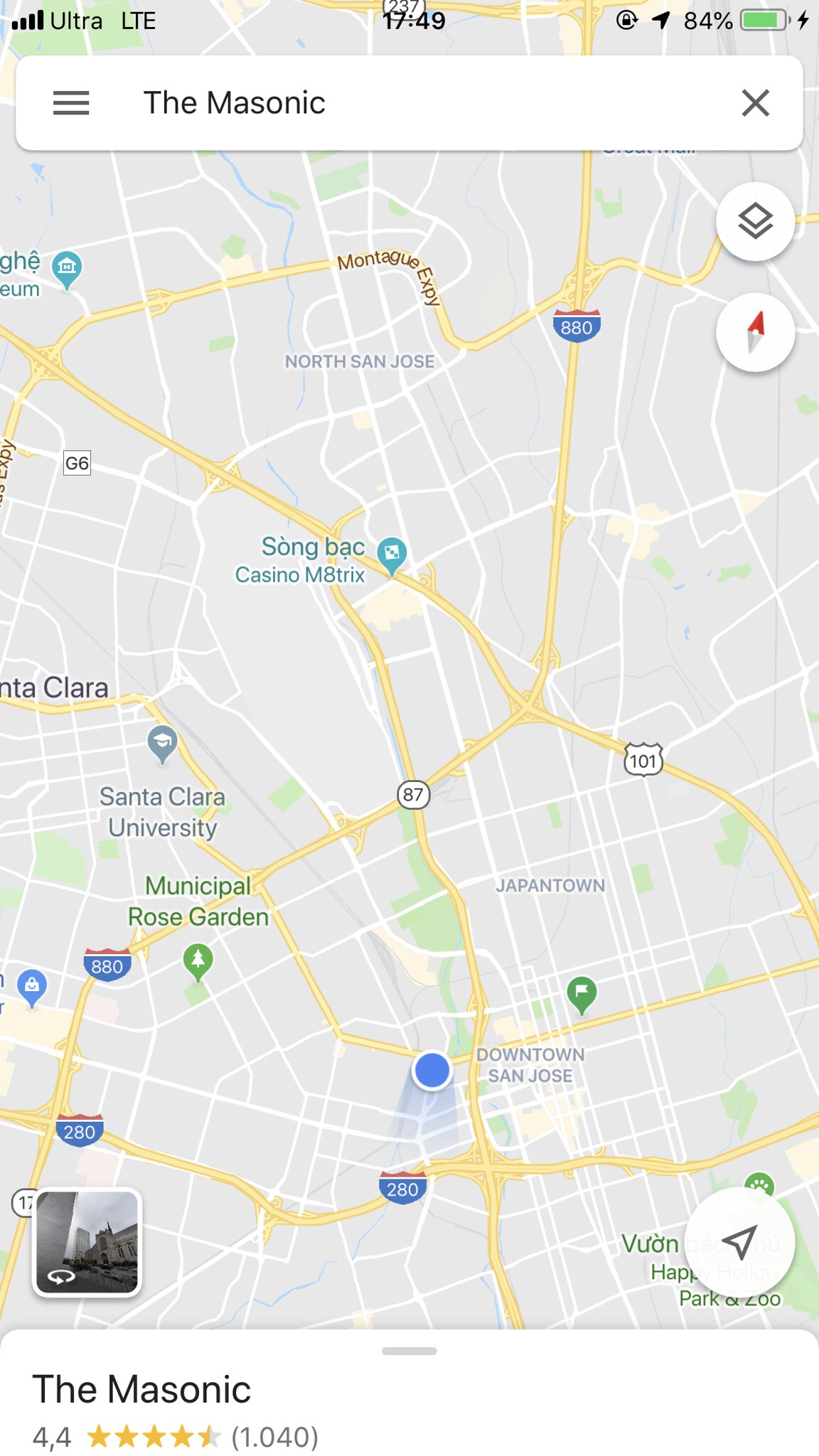This image is a screenshot of a map from a smartphone, displaying the area around Interstate 880 and nearby highways. The map is centered on "The Masonic," which is a location rated 4.4 stars with 1040 reviews, as indicated in text at the bottom. Above the map, there is a search bar with the entry "The Masonic" highlighted in white. 

In the top left corner of the screen, various status icons are visible: four bars indicating cellular signal strength with "Ultra LTE" text, the time "17:49," a battery icon showing 84% charge with a lightning bolt indicating charging, a lock screen icon, and an arrow icon.

Several landmarks and routes are marked on the map, including Interstate 880 displaying a north-to-southwest trajectory, Route 101, and Highway 87. Notable locations such as Santa Clara University, the Municipal Rose Garden, Downtown San Jose, Japantown, and Montague Expressway are clearly labeled. 

Overall, the screenshot provides a comprehensive overview of the area surrounding "The Masonic," complete with navigational routes and significant local points of interest.